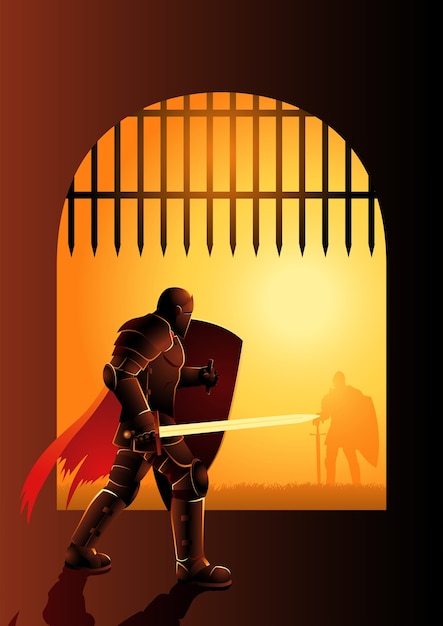The illustrated image depicts a dramatic scene between two knights, shrouded in shadows and mystery. The foreground knight, clad in dark armor, strides purposefully forward from a dimly lit cave or castle interior, his tattered red cape trailing behind him. He holds a gleaming silver sword in one hand while his other arm bears a sturdy shield. Above him, the grates of a gate hover mid-rise, suggesting he is just stepping out. The intense light of a bright orange sun spills into the scene from outside, creating a stark contrast that renders the second knight, standing in the distance, into a mere silhouette. This second knight, also armored and holding a shield, braces his sword against the ground, giving an impression of waiting — though whether as an ally, foe, or a figure of unknown significance remains unclear. The interplay of light and shadow, along with the position of the knights, imbues the image with a sense of suspense and questions about the impending interaction between the two figures.